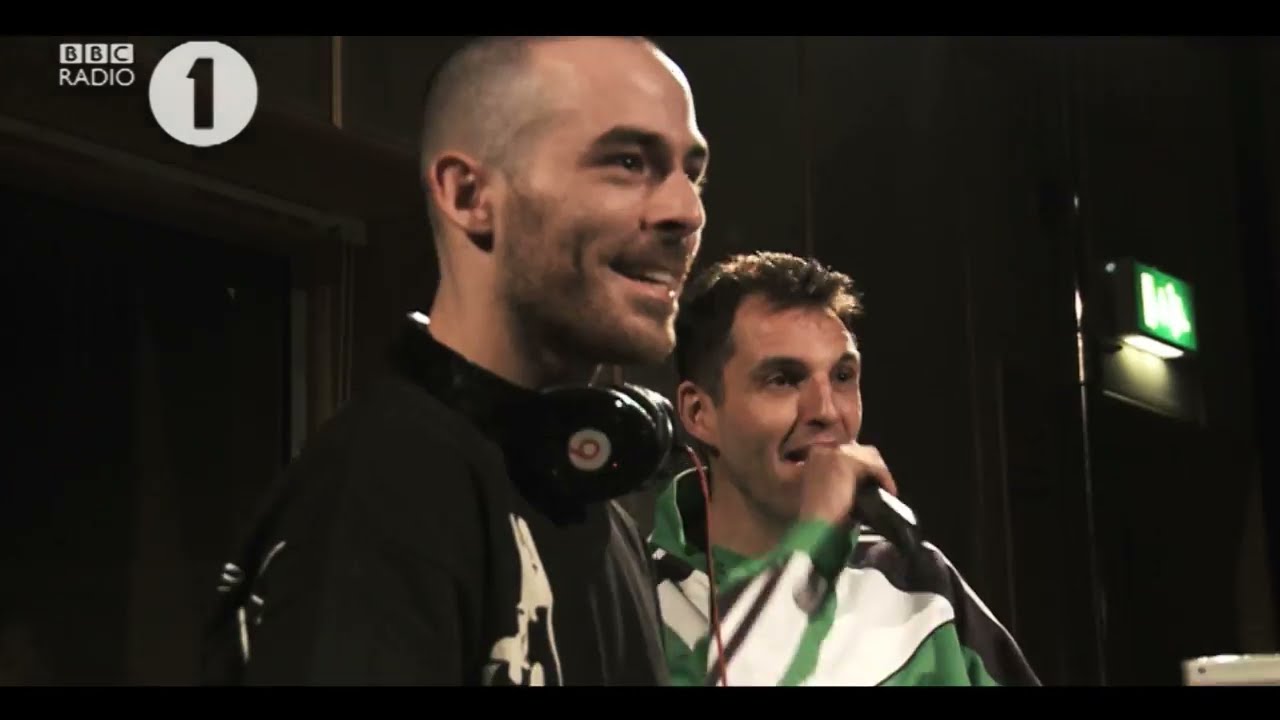The image depicts a recording studio, likely from a radio show, with the notable presence of Nicki Minaj giving an interview. She is seated in front of multiple microphones, identifiable by the "BBC Radio 1 Extra" label on the microphone cover. Nicki has long blonde hair, likely a wig, and is wearing a black leather jacket. Over-the-ear headphones are snugly fitted on her head, and she appears to be talking animatedly, her right hand in motion, creating a slight blur. Her makeup is striking, with long eyelashes and pink lipstick.

Nicki is positioned on the right half of the image, while the left half showcases various studio equipment. The workspace includes two computer keyboards, two computer mice, a pair of black sunglasses, and a nearly empty clear plastic water bottle. The setting is replete with color accents including shades of yellow, white, black, gray, red, blue, and pink, but overall dominated by black elements. Another individual, possibly a producer or co-host, is partially visible next to Nicki. This person is wearing a blue t-shirt and has a bracelet on their right wrist along with a ring on their pinky finger. The studio ambiance is cozy yet filled with professional broadcasting gear, capturing the intensity and engagement of a live radio interview.